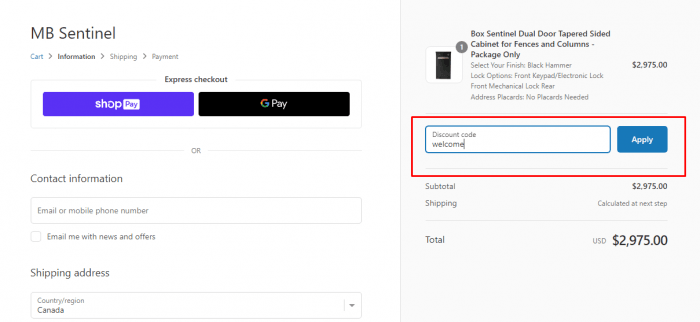Screenshot Description: Checkout Page for MB Sentinel on E-commerce Website

On the left section of the page, the background is predominantly white. The top left corner features the brand name "MB Sentinel" prominently. Beneath that, there are navigation indicators in sequence: "Cart Information," "Shopping," and "Payment." Centered on the page below these indicators is the label "Express Checkout" in bold black font.

Directly under "Express Checkout," there are two prominent action buttons for payment methods. The button on the left is purple and includes the text "Shop Pay" displayed in white. Next to it on the right is a black button with the "Google Pay" logo; the "G" is colored in green, red, yellow, and blue, while the word "Pay" is in white.

Below these buttons, the page prompts for "Contact Information," allowing the user to input an email or mobile phone number. Following this is a section for the "Shipping Address," which includes an option to select the country.

On the right section of the page, there is a summary of the selected product, described as a "Sentinel Dual Door Tampered." A picture of the product is provided, depicting a white box containing a black object. Below the product description is a box for entering a discount code, labeled "Welcome." 

This discount input area has a red outline and a blue, rounded-edge button labeled "Apply" on the right side. Below this section, the price breakdown is shown, including the subtotal, shipping, and the final total cost prominently displayed as $29,975.